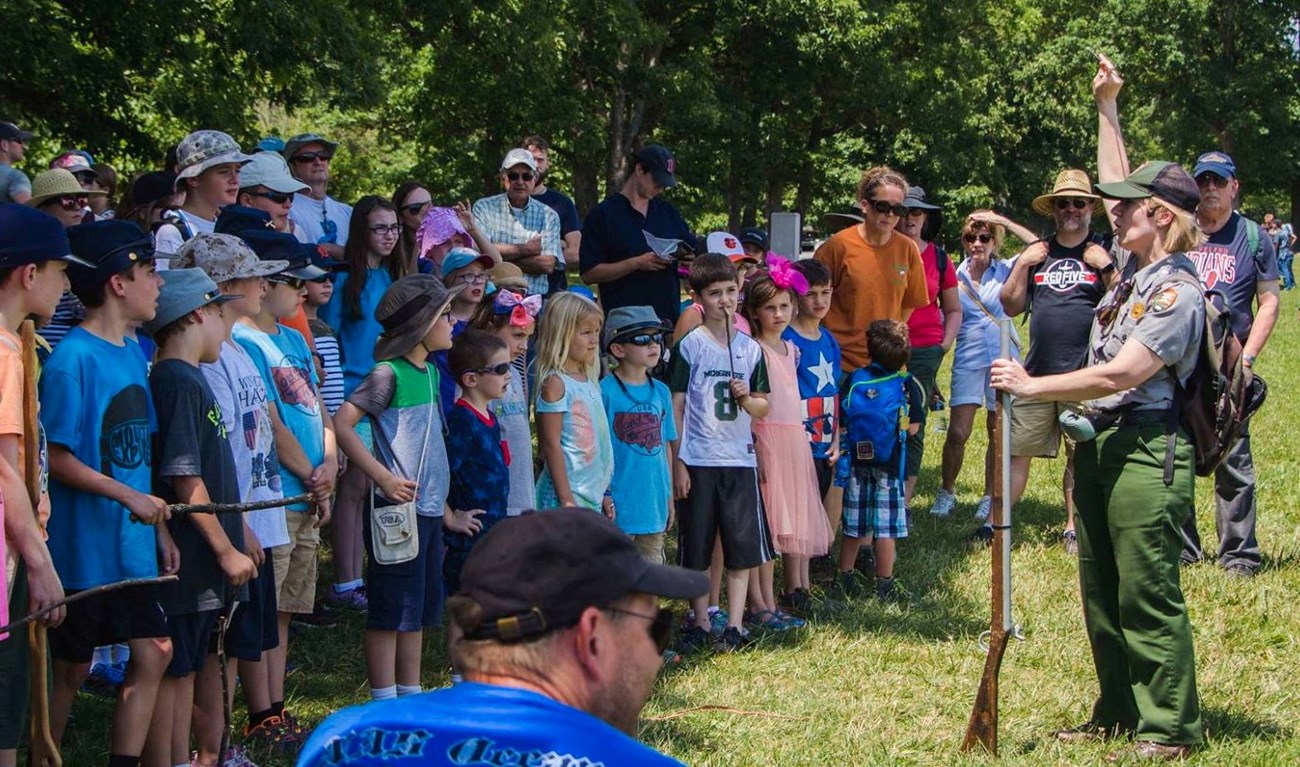This high-quality color photograph, taken outdoors during the summer, captures a large group of children and their parents attentively listening to a woman in a uniform. The woman, who appears to be a park ranger or scout leader, stands to the left of the crowd. She is distinguished by her green pants, shirt adorned with patches, a green baseball cap, and a backpack. Her right arm is raised, and with her left hand, she steadies a long rifle or musket, its butt resting on the ground. The children, primarily in shorts and short-sleeved shirts, some wearing dresses, hats, and sunglasses, stand in a line facing her. The parents are scattered among the children, all focusing on the woman. The scene is set against a backdrop of lush green trees, with everyone standing on vibrant green grass. In the foreground, a man is seated, wearing a black ball cap, sunglasses, and a blue shirt.